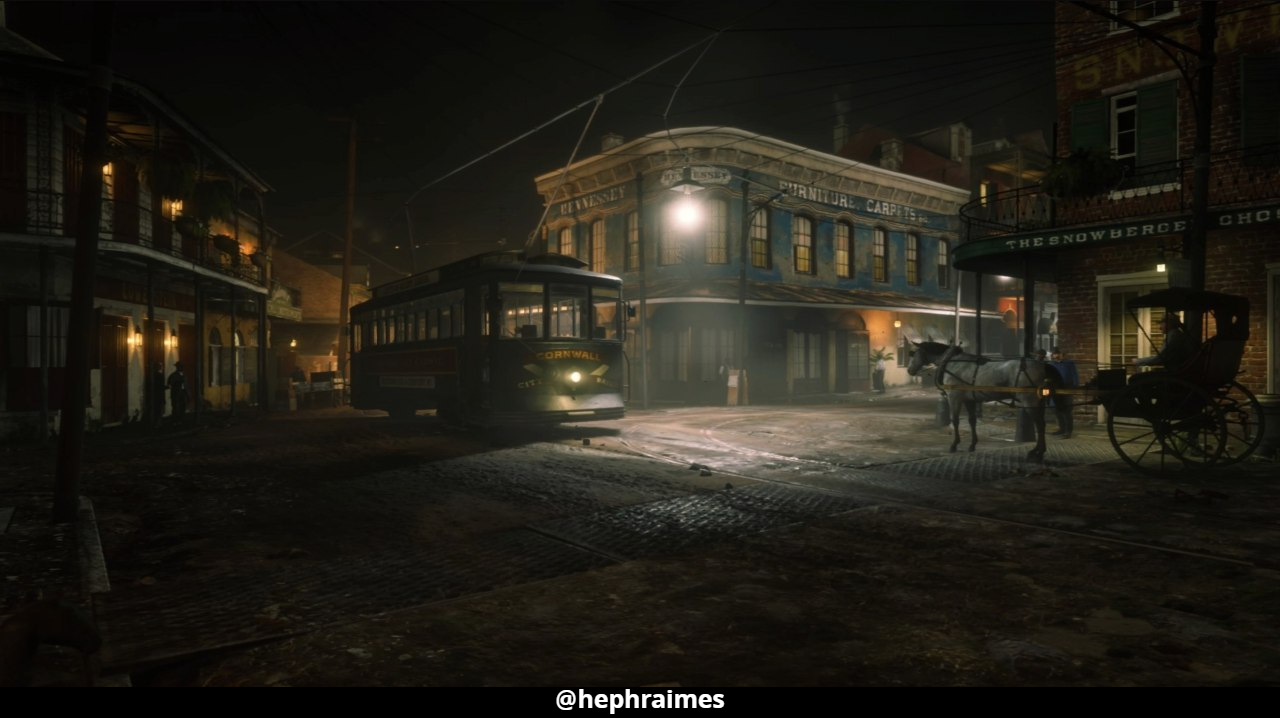A nighttime scene unfolds in this detailed outdoor image. The dark sky looms overhead, casting an atmosphere of quiet and serenity. At the very bottom of the image, the text reads "Hephreimes," lending a sense of place to the scene. The ground is cobblestone, adding a historical layer to the environment. On the right side, a majestic white horse is hitched to a black carriage with large, round wheels, capturing a moment frozen in time. On the left, a tram with multiple windows, each dimly illuminated, waits in the darkness. It is connected to an overhead wire for power and a bright headlamp at the front pierces the gloom. Adjacent to the tram, a balcony adorned with lights provides additional illumination. Dominating the center is a grand, corner building, its architectural grandeur highlighted by a light at the top. The overall imagery harks back to an old-timey setting, rich in historical ambiance and captivating details.